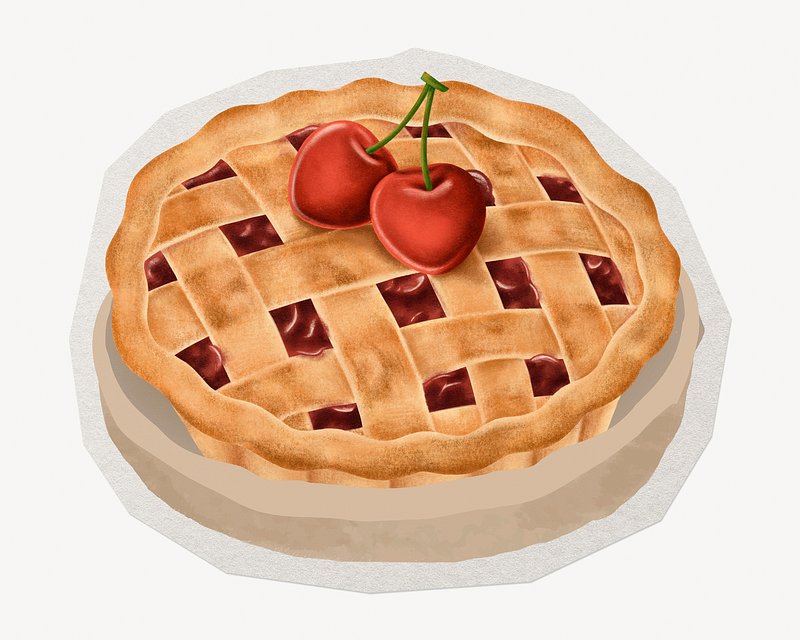This image depicts a detailed drawing of a cherry pie, reminiscent of advertising artwork from the 1950s or 60s. The pie features a golden brown lattice crust with peeks of vibrant red cherry filling shining through. On top of the lattice crust, two prominently large maraschino cherries with green stems are placed, emphasizing the cherry flavor of the pie. The pie sits on a beige plate, which rests against a subtle grayish background, creating a slight shadow effect. The entire scene is set against a clean white backdrop, highlighting the pie's detailed and nostalgic appearance.